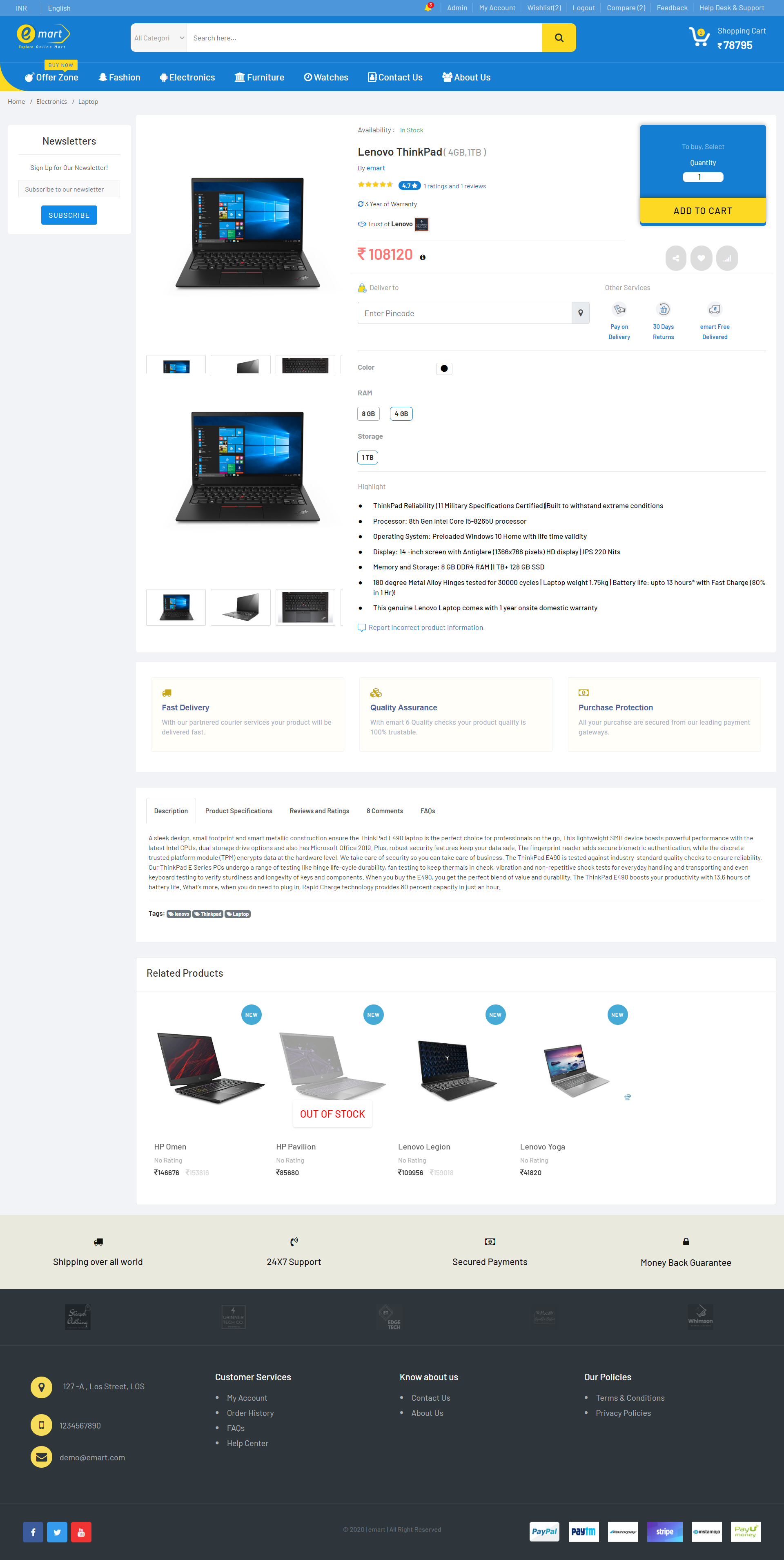The image features a blue background with several elements organized across it. At the top, there is a dark blue box accompanied by a yellow circle in the upper left corner, with a small yellow triangle also in the left corner. Below this, a prominent white search box with yellow accents on the edges is visible, along with a yellow button and a shopping cart icon displaying some numbers.

To the side, the blue background continues, and there is a white box containing a blue button. Adjacent to this, there is a dropdown menu with a white background. Two computer listings are displayed, each featuring prices marked in pink. Nearby, a small blue box with yellow at its base can be seen. Light blue lines and additional text appear sporadically.

Further down, another white box displays blue print. There are also images of four small laptops, each marked with a blue circle in the top right corner. Below these, a gray box contains various icons, and at the very bottom, a black box hosts three yellow circles. The lower section of the image includes icons for Facebook, Twitter, and other social media platforms, along with what appears to be a charge card icon.